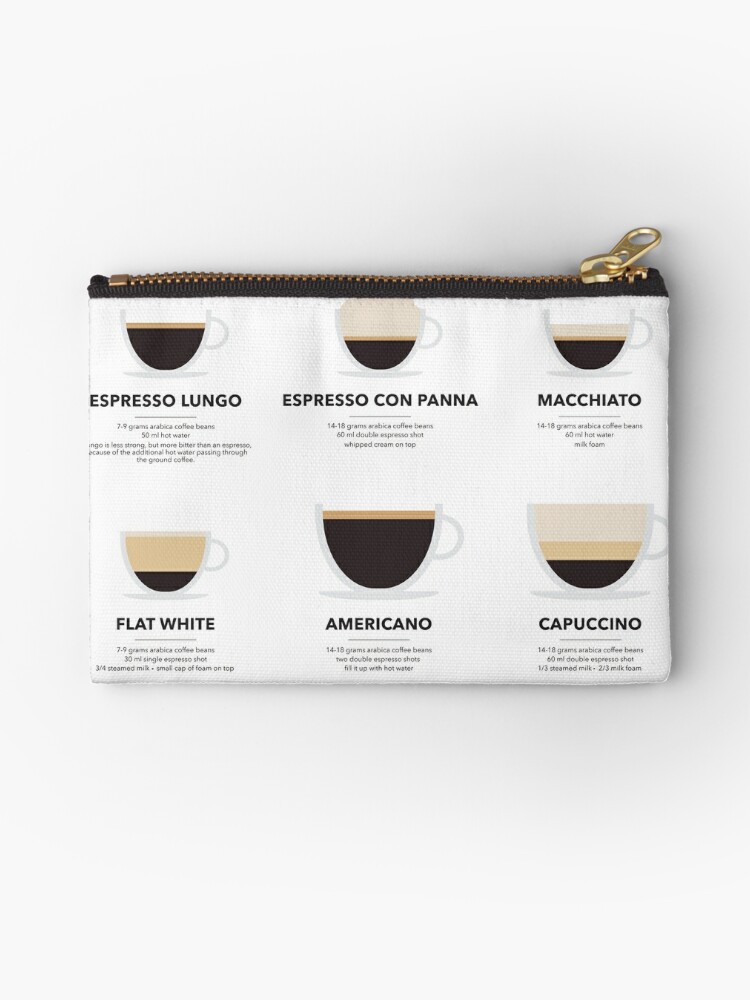This photo, in portrait orientation, features a detailed image of a small, rectangular coin purse or clutch, predominantly white in color with a dark brown trim around the top. The purse boasts a golden zipper attached to a black fabric strip, with the brass zipper pull positioned on the right side. The front of the purse is adorned with a design featuring six different types of coffee cups, arranged in two horizontal rows of three. Each cup is filled to varying levels and is labeled in black text with the corresponding coffee type: starting from the top left, there is an Espresso Lungo, followed by Espresso Con Panna, and Macchiato. On the bottom row from left to right, the sequence continues with a Flat White, an Americano in the center, and a Cappuccino. This realistic, representational photograph captures the intricate details of the purse's design, including the handles of the coffee cups positioned on the right, set against a light gray background, suggesting an emphasis on product photography.